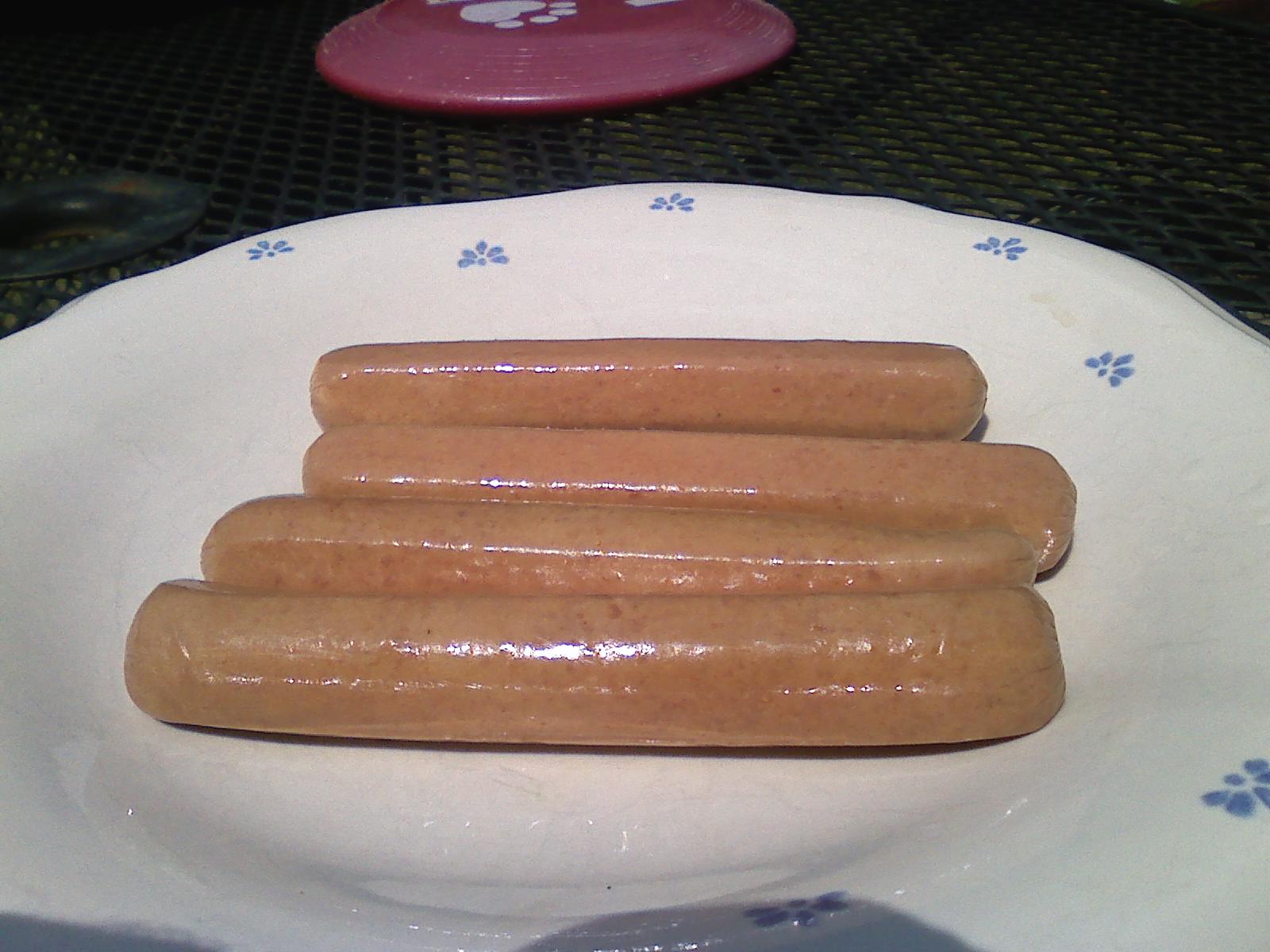The photograph depicts an intricately detailed scene at a house, featuring four uncooked hot dogs arranged horizontally on a white dinner plate that sinks in the center. The plate is adorned with a delicate blue floral pattern along its edge. The hot dogs are a light brownish-pink with darker flecks, glistening as they likely reflect light due to residual brine. The plate is set on a black metal mesh table, which creates a textured backdrop. At the top of the image, a red frisbee with ridges around its circumference and stamped with a white paw print rests partially over the plate. Also visible towards the left is a ring, likely part of the table designed for placing an umbrella. Shadows add depth to the scene, emphasizing the rich, contrasting colors and textures.